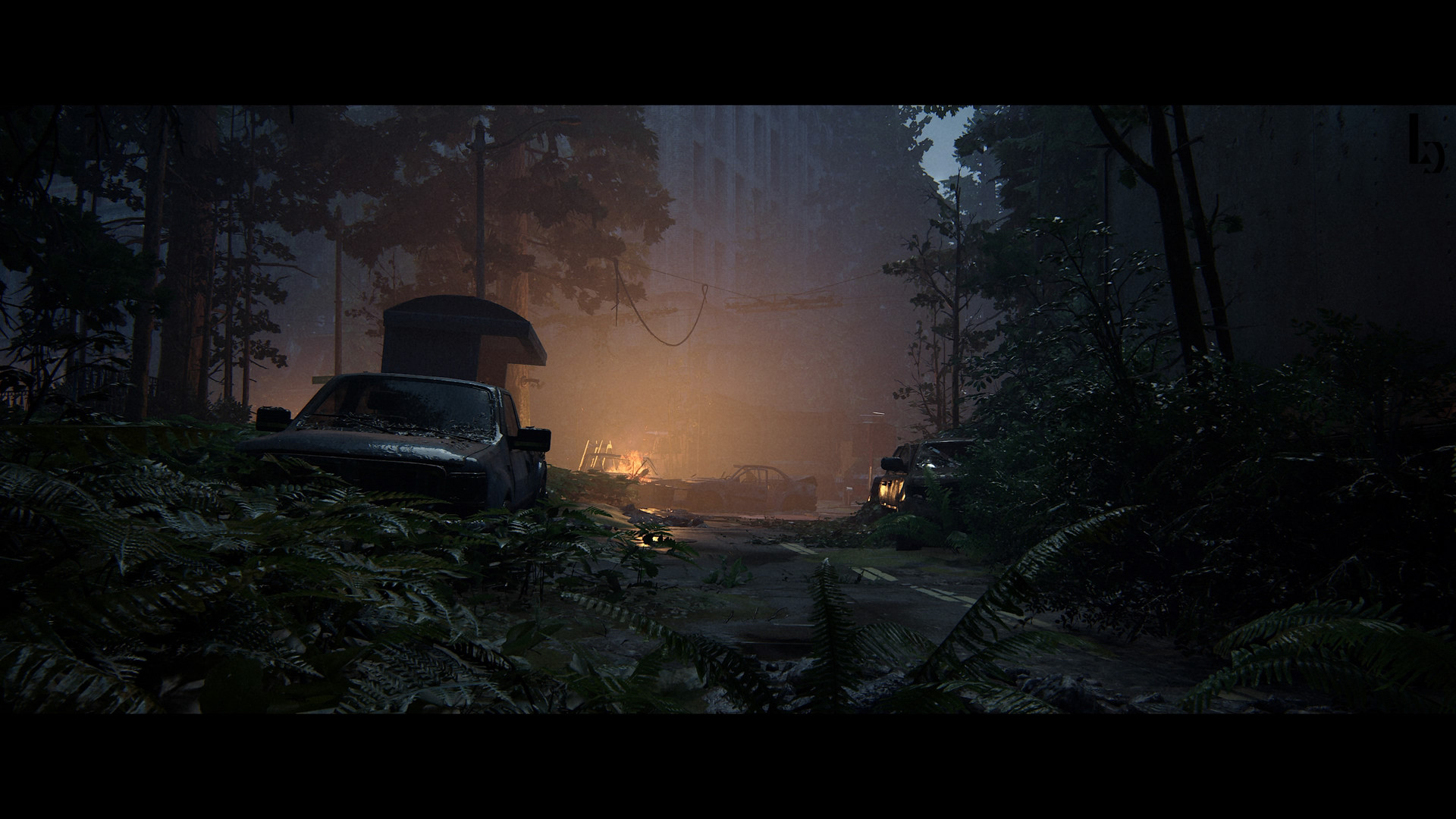In this captivating twilight scene set in a dense forest, the dim natural light accentuates an atmosphere of tranquil mystery. The old, overgrown road, bordered by lush green ferns and sporadically spaced young trees, weaves through the heart of the wilderness. To the left, a weathered gray pickup truck stands quietly among the foliage, a relic of a bygone era. On the right, in the background, another abandoned vehicle sits ensconced in the landscape, adding to the sense of abandonment. Amidst the trees, a source of warm yellow light glows softly, perhaps a small fire or an enigmatic luminescence, casting a gentle glow on the surroundings. In the distance, the tops of gray apartment buildings or a multi-story structure peek through the treetops, juxtaposing urban life against the untamed nature. The scene encapsulates a serene blend of human presence and the enduring spirit of the forest.